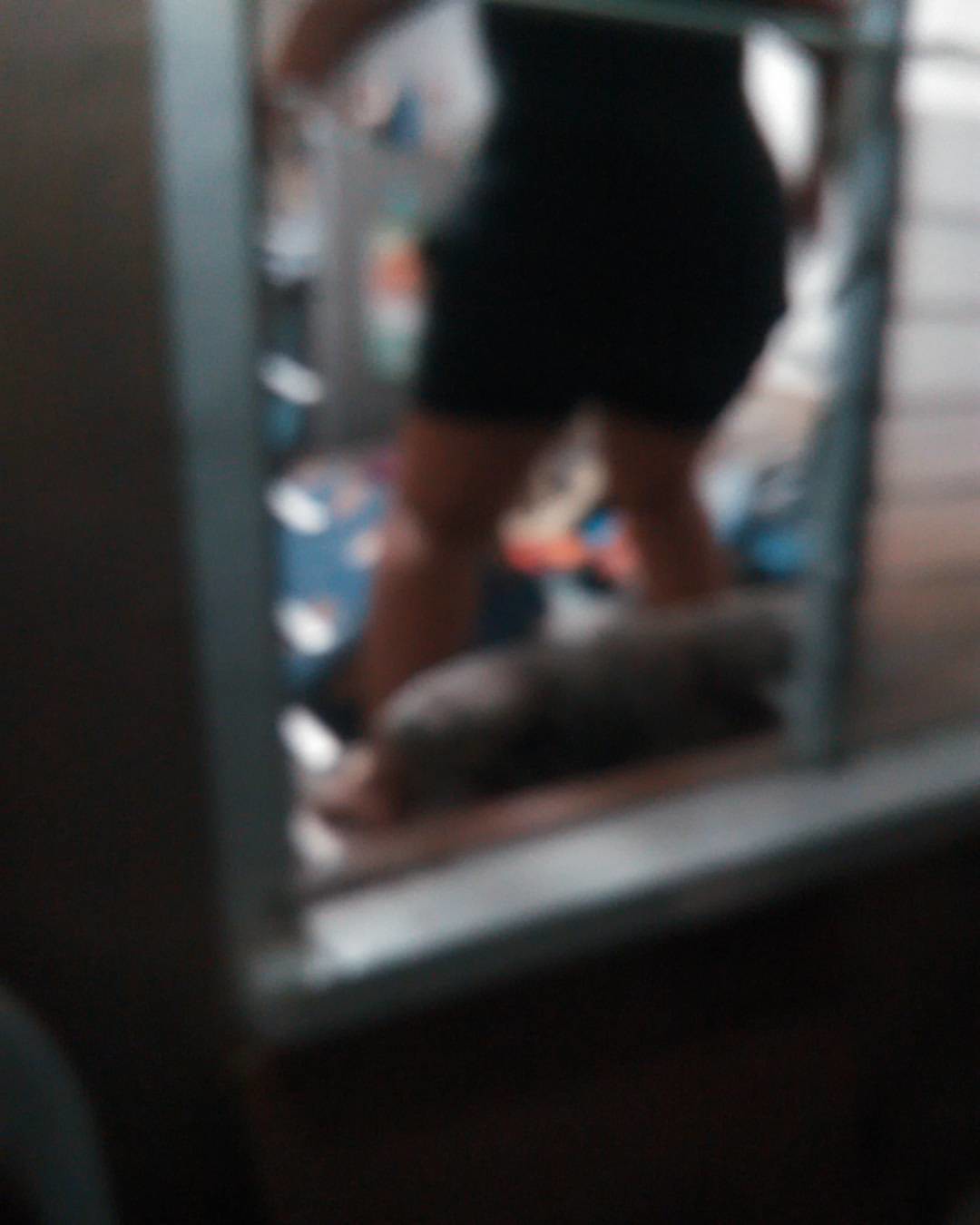The image depicts a very blurry scene shot from outside a house, looking through a white-trimmed window with a brown wooden frame, possibly made from wooden decking. Inside the room, a person, likely a woman, is visible standing. She appears to be wearing blue shorts and a blue t-shirt. Her arms are raised high, and she stands amongst colorful, indistinct items on the floor, potentially bean bags or children's toys. The room is lit from within, creating a stark contrast to the apparent nighttime setting outside. An additional slatted glass window is slightly to the right and remains intact, while a broken slatted glass window is visible near the top left edge of what seems to be a gray couch. The far wall inside the room features a large black TV. The house's exterior is primarily brown wood, with some descriptions suggesting an off-white or light gray-blue hue.